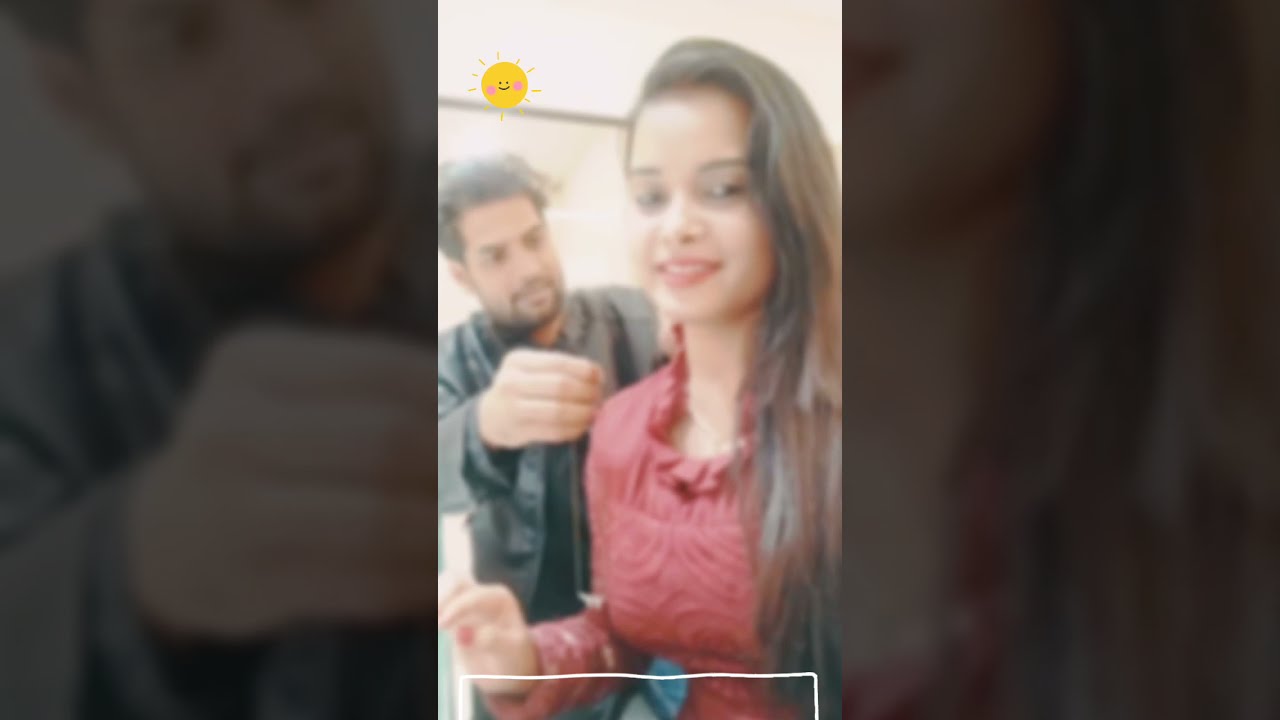The image is composed of three vertically aligned panels with the central panel highlighted and the side panels darkened and zoomed-in close-ups of the center photo. In this central panel, we see a slightly blurred image of a woman and a man, both appearing to be of Indian descent. The woman in the foreground is wearing a long-sleeved, intricately designed red blouse with a ruffled neck border. She has long brown hair that falls mostly over her left shoulder and is looking down and to the left. She appears to be holding the camera out of view with her left hand and is captured smiling slightly.

Behind the woman, a man with black hair and a thin stubbled goatee is seen reaching out towards the woman’s shoulder with his right hand. He is wearing a black leather jacket and is looking directly at the woman, rather than the camera. Above his head, there is an emoji of a smiling sun with blushed cheeks, adding a whimsical touch to the scene. The overall setting seems to be indoors, possibly illuminated by sunlight, hinting at large windows or a well-lit room with a white wall and ceiling in the background.